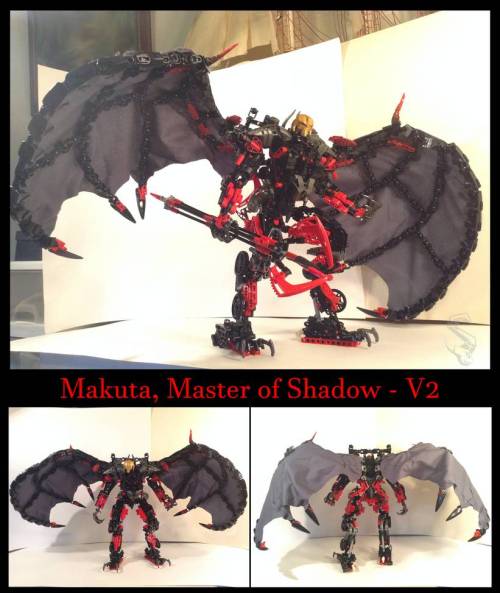The image showcases an intricately assembled action figure named Makuta, Master of Shadow-V2, prominently displayed against a black background. The figure, reminiscent of a Lego Technic or a customized toy akin to a Gundam model, is constructed primarily in black with accents of red, yellow, gray, and gold. Makuta features large, dragon-like wings with black or gray felt creating the wing effect, adding to its menacing appearance.

The figure is armed with a red and black weapon and is detailed with significant body armor, enhancing its complex and mechanical look. The head stands out with its bright yellow color, contrasting with the darker hues of the body. The top portion of the image displays a large profile view of Makuta, while the bottom half showcases two smaller images, presenting the figure from the front and the back. Text in red prominently reads "Makuta, Master of Shadow-V2" between the images, likely indicating a second version or variation of the model. The image, likely intended for collectors or enthusiasts, highlights the detailed craftsmanship and elaborate design of the action figure.